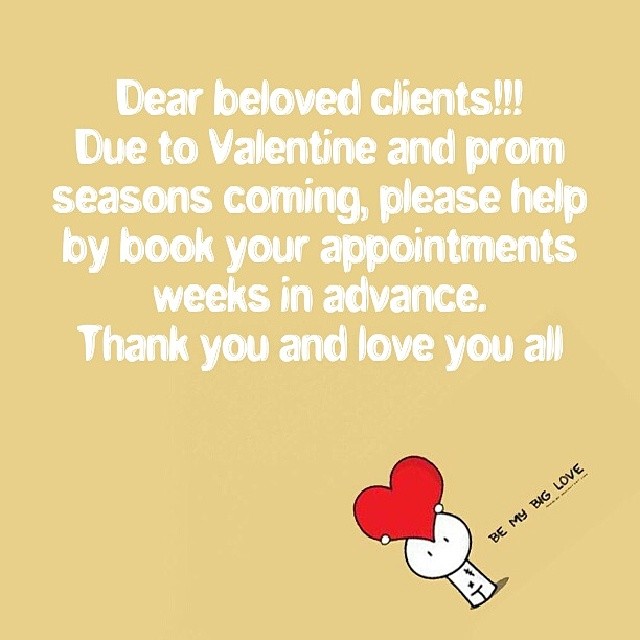This vertical rectangular announcement poster features a beige background that graduates from a darker tone at the top to a lighter shade towards the bottom. The white-centered text spans about six lines and reads: 

"Dear Beloved Clients!!! Due to Valentine and prom seasons coming, please help by booking your appointments weeks in advance. Thank you and love you all."

Beneath the text, in the bottom right corner, is a playful cartoon design—a small character, depicted with a simple circle for a head, two dots for eyes, a rectangle for the body, and holding a large red heart where the face would be. The heart has a black outline and hovers over the character's head. Next to this quirky figure, the phrase "BE MY BIG LOVE" is written in all capital black letters, with "BIG LOVE" underlined for emphasis. This charming visual and heartfelt message appears to be posted within a store to alert and encourage clients to schedule their appointments well in advance of the busy Valentine and prom seasons.